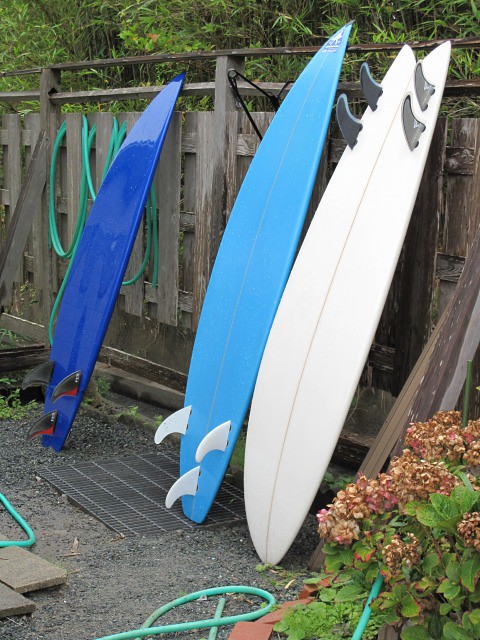This outdoor photograph captures a backyard scene featuring three surfboards propped up against a wooden fence composed of vertical slats. The background boasts lush greenery from trees, adding a natural touch. At the foot of the scene is a mix of dirt and gravel, interrupted by a metal grate. A green garden hose snakes through the gravel and dirt, both circling around the yard and looping through some brush in the lower right corner, where a hydrangea bush with green leaves and dead brown flowers stands out. Leaning against the fence on the left is a royal blue surfboard, distinguishable by the three brown shark-fin inserts at its base. Next to it, a light blue surfboard, Carolina blue in shade, also stands upright, showcasing three white fins at the bottom. Finally, furthest to the right, a white surfboard rests against the fence, positioned with its tip down, revealing four small fins at the tail.